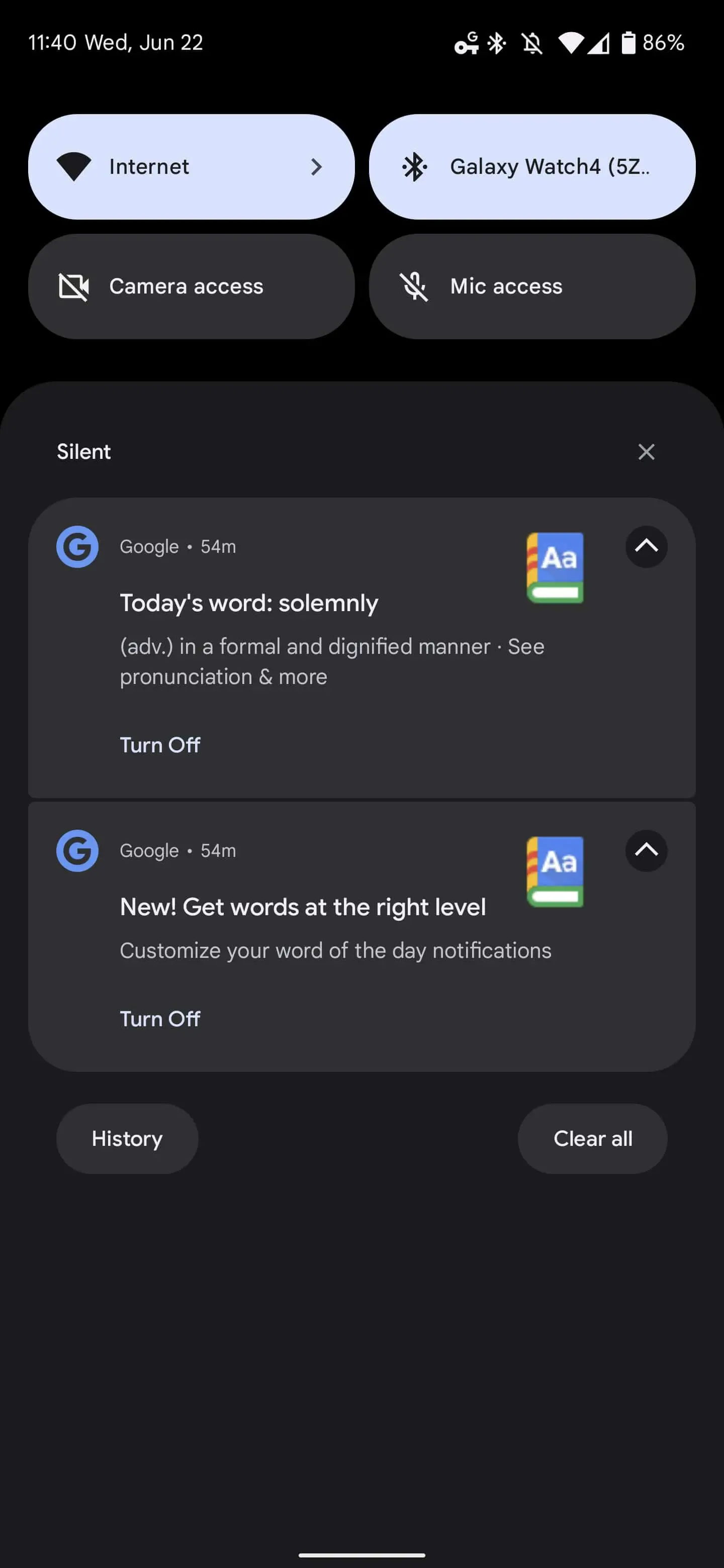The image is oriented in a vertical rectangle with the longer side extending from top to bottom. The background is entirely black, presenting a stark contrast to the content in the foreground. 

In the top-right corner, there's a snippet resembling a smartphone interface. It displays the time "11:40," the date "Wednesday, June 22," and a series of status symbols on the right. The symbols include an unidentified icon, a Bluetooth symbol, a muted bell icon, a full Wi-Fi signal, a cellular signal with 3 out of 4 bars, and a battery indicator showing an 86% charge.

Beneath this information is a set of interface options, beginning with an oblong, light blue box labeled "Internet" alongside a Wi-Fi symbol. To the right, another oblong box features the Bluetooth symbol and the text "Galaxy Watch 4." Below these, two additional oblong boxes appear, both black with white text. The first reads "Camera Access" accompanied by a camera icon with a line through it, indicating restricted access. The second reads "Mic Access," with a similar crossed-out microphone icon indicating restricted microphone access.

Further down the image, the section labeled "Silent" is on the left, with an "X" on the right. Below this area, there are two more sections. One shows a blue circle with a black "G" inside and the text "Google, 54M." The final section provides the "Word of the Day" as "solemnly."

This meticulous arrangement of elements on a dark background suggests a detailed user interface, likely from a smartphone, complete with various important notifications and controls.